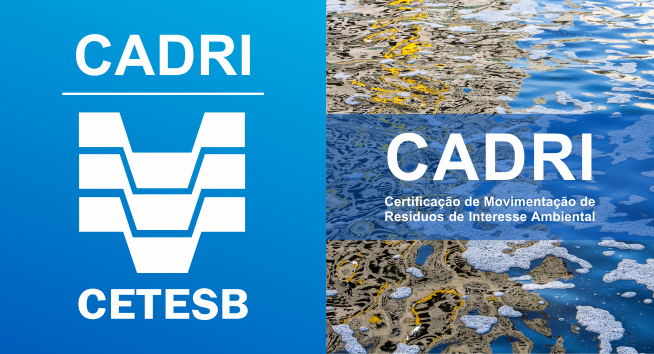The image features a corporate advertisement divided into two almost square sections. On the left, the background is blue and prominently displays the company name "Cadri" in large white letters. Below the name is a corporate logo consisting of three identical symbols aligned horizontally, with the text "C-E-T-E-S-B" underneath. On the right, there's a photo of a body of water covered with algae or a film possibly resembling oil. Superimposed on this image, "Cadri" appears again in white letters, accompanied by a tagline in a foreign language, potentially Spanish or a related language. The full tagline reads: "Certifico de Movimento de Residuos de Interesse Ambiental." The overall color palette includes shades of blue, white, brown, yellow, and black, and the layout suggests a professional design likely intended for a company website.